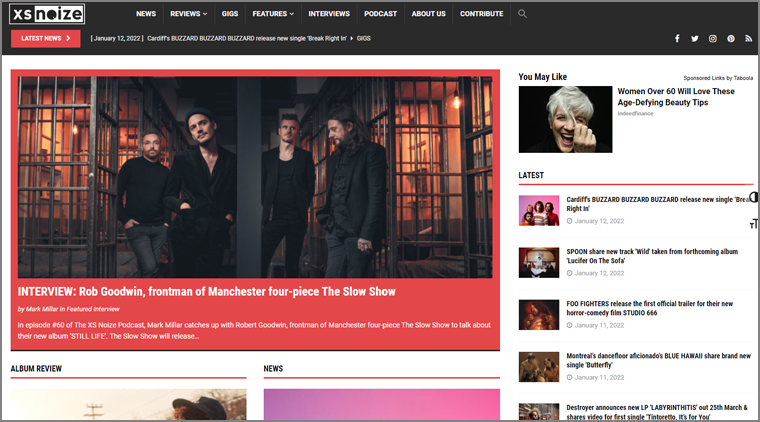In this detailed image of the XS Noise website, the top-left corner prominently displays the website's name, "XS Noise," styled as "XS NOIZE." Just below the website name is a bold red rectangle with the text "Latest News." 

The navigation menu spans horizontally at the top of the page, showcasing white category names on a black background. The categories, listed from left to right, are: "News," "Reviews," "Gigs," "Features," "Interviews," "Podcasts," "About Us," and "Contribute." Adjacent to these categories on the far right is a search icon.

In the bottom right corner of the header, there are icons for various social media platforms, including Facebook, Twitter, and Instagram, along with two additional, unrecognized icons, all rendered in white.

Below the header, the main background color transitions to white. Dominating this section is a large red square image featuring four band members positioned near illuminated jail cells with a distinct orange lighting. Beneath this visual, text reads: "Interview with Rob Goodwin, frontman of Manchester Four Piece, The Slow Show," accompanied by some smaller white text underneath.

Further down, two categories are highlighted: "Album Review" and "News," each underlined with a red line.

On the right-hand side, there's a section titled "You May Like" followed by an advertisement with the text: "Women Over 60 Will Love These Age-Defying Beauty Tips."

Below the advertisement is a "Latest" section, presenting five selectable options displayed in black text, each accompanied by a corresponding image to the left.